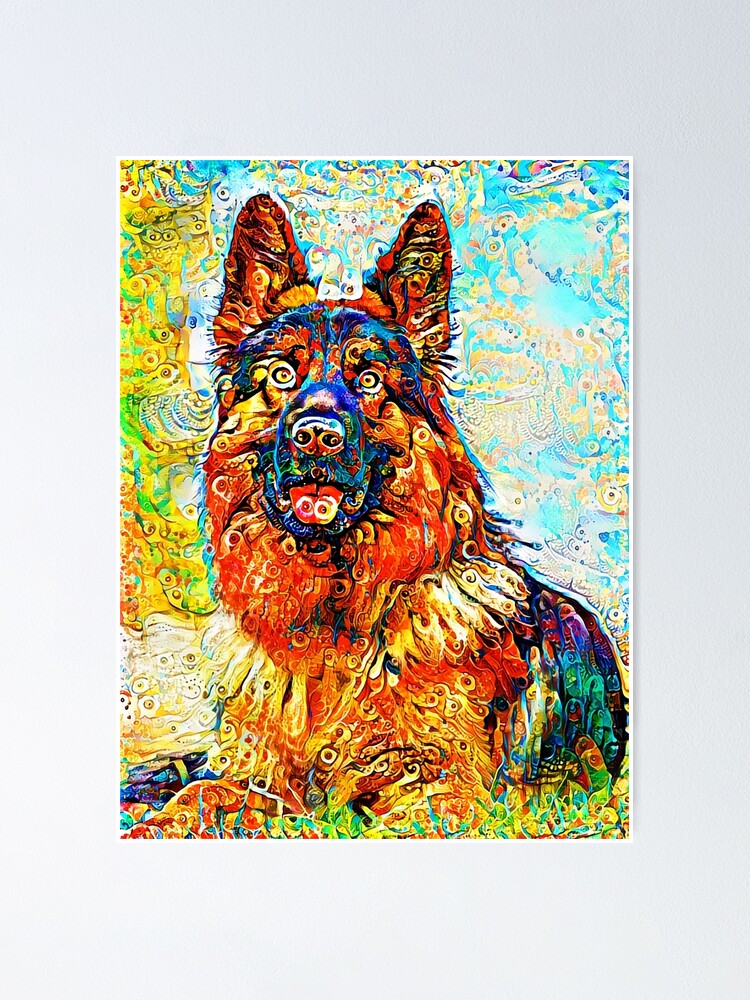This poster-sized painting, mounted on a light gray wall with a narrow white frame, features a German Shepherd in a vibrant, impressionist style. The painting captures the dog sitting down, its head and chest dominating the frame, and it looks directly at the viewer with golden eyes wide open and a panting mouth revealing a pink tongue adorned with both yellow and pink swirls. The artwork is characterized by a multitude of intricate swirls and swooping designs in neon colors, giving it a psychedelic, almost trippy feel. The German Shepherd's coat features a blend of colors with a darker blue muzzle and crown, golden-orange face, ears, chest, and accents of green, black, red, and orange that almost evoke a peacock feather-like composition. The background, divided into two distinct parts, features a lively blue sky with white and yellow swirls and subtle red dots on the right, juxtaposed with a yellow section on the left, adorned with green, black, and red swirls, possibly suggesting a tree. The bottom of the painting hints at grass, and overall, the piece conveys a bright and cheerful demeanor of the dog against a vividly abstract and colorful backdrop.